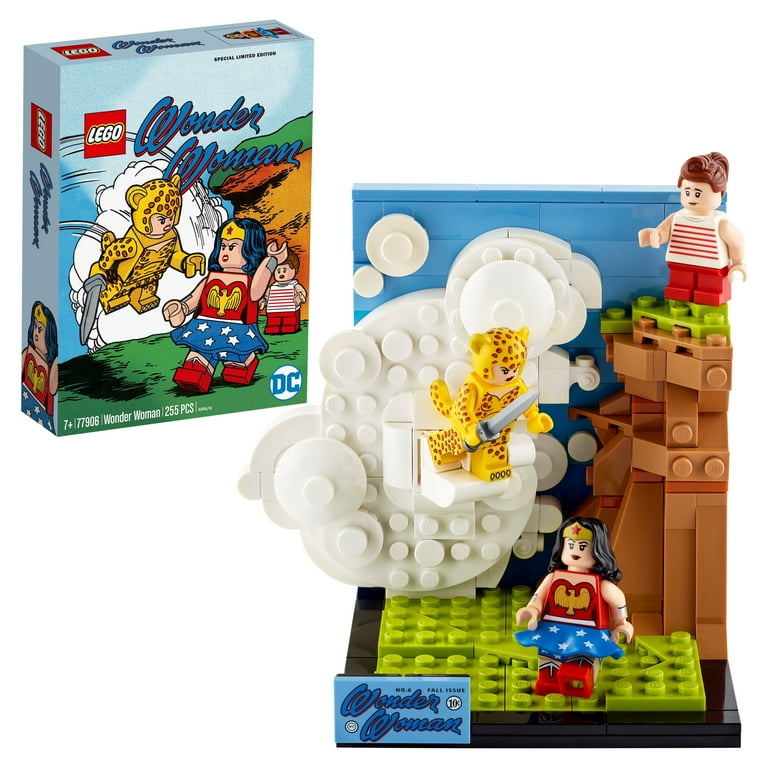This detailed product image showcases an assembled Lego Wonder Woman kit alongside its packaging on a white background. The image on the right features the completed Lego scene, where Wonder Woman, wearing her iconic blue star-spangled skirt, white top with an eagle design, and gold headband with a red star, stands on a green surface. In front of her is a small plaque labeled "Wonder Woman." Behind her is a cloudy formation with a figure dressed in a leopard costume wielding a knife, representing Cheetah, and to the right, a tree with a Lego figure wearing a white shirt with horizontal red stripes perched in its branches. The packaged box, depicted in the upper left, includes a cartoon image of Wonder Woman facing off against Cheetah and the set details, such as the Lego logo, "Wonder Woman," age recommendation "7+", set number "77790," "255 pieces," and the DC branding.